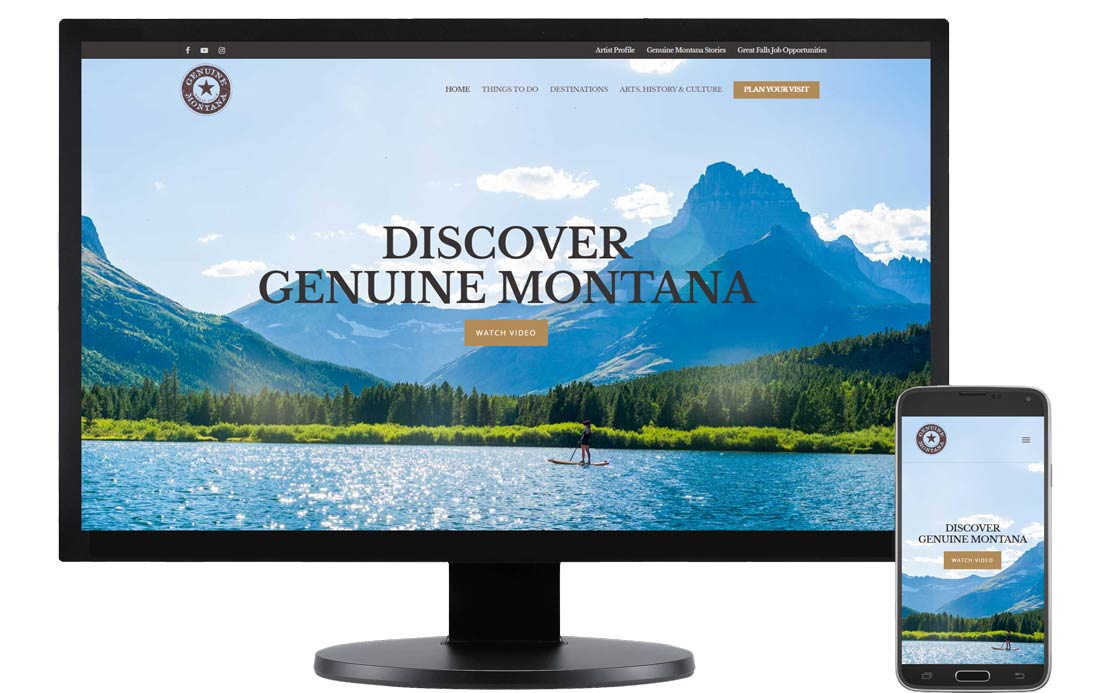Here is a cleaned-up and detailed caption for the image:

---

The image showcases both a computer screen and a smartphone displaying matching websites for "Discover Genuine Montana." The central focus on both devices is the text "Discover Genuine Montana," positioned prominently over a stunning background. The background features a picturesque mountainous area with a serene, blue lake in the foreground. A person is seen paddleboarding, standing on their board in the middle of the glistening water under abundant sunlight. Surrounding the lake, there are tall grasses and fir trees, which ascend a hill to the right. In the distance, taller bluish mountains are visible beneath a clear blue sky dotted with a few clouds that allow sunlight to filter through beautifully.

Beneath the "Discover Genuine Montana" text, there's a gold button with white text that reads "Watch Video." In the top-left corner of the screen, a circular logo with a brown ring and blue center catches the eye. The logo, which reads "Genuine Montana" around the ring, features a centered brown star.

To the right of the logo, a navigation menu consists of brown text in all caps: "HOME," "THINGS TO DO," "DESTINATIONS," "ARTS," "HISTORY," and "CULTURE." There's also a gold button with white text reading "PLAN YOUR VISIT." At the very top of the screen, a header includes icons for Facebook, YouTube, and an unidentified platform on the left. On the right, it lists "ARTIST PROFILE," "GENUINE MONTANA STORIES," and "GREAT JOB OPPORTUNITIES" in white text.

The smartphone screen mirrors this display but with some adjustments to fit the smaller screen. It features the same central image and text but replaces the top words with a three-line menu icon at the top right corner.